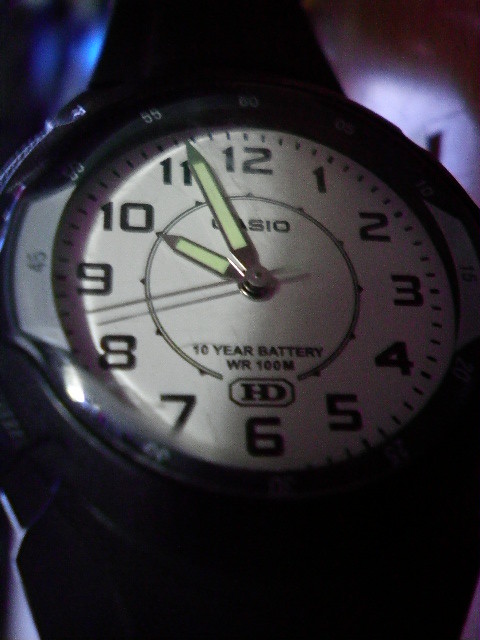This striking close-up of a wristwatch captures the contrast between light and shadow as they split the image down the middle. The left side is bathed in sunlight, highlighting the watch's details, while the right side resides in shadow, adding depth and drama to the scene. The watch features a clean, white face adorned with black numerals and sleek silver hour and minute hands that appear to have glow-in-the-dark strips. A polished silver second hand glides over the surface. Positioned just below the 12 o'clock marker, the Casio logo stands out clearly. Near the 6 o'clock marker, the text "10-year battery WR100M" is featured prominently, with "HD" boldly displayed underneath it. Encasing the watch is a black bezel, complemented by a matching black wristband that adds to the overall classic and versatile design.